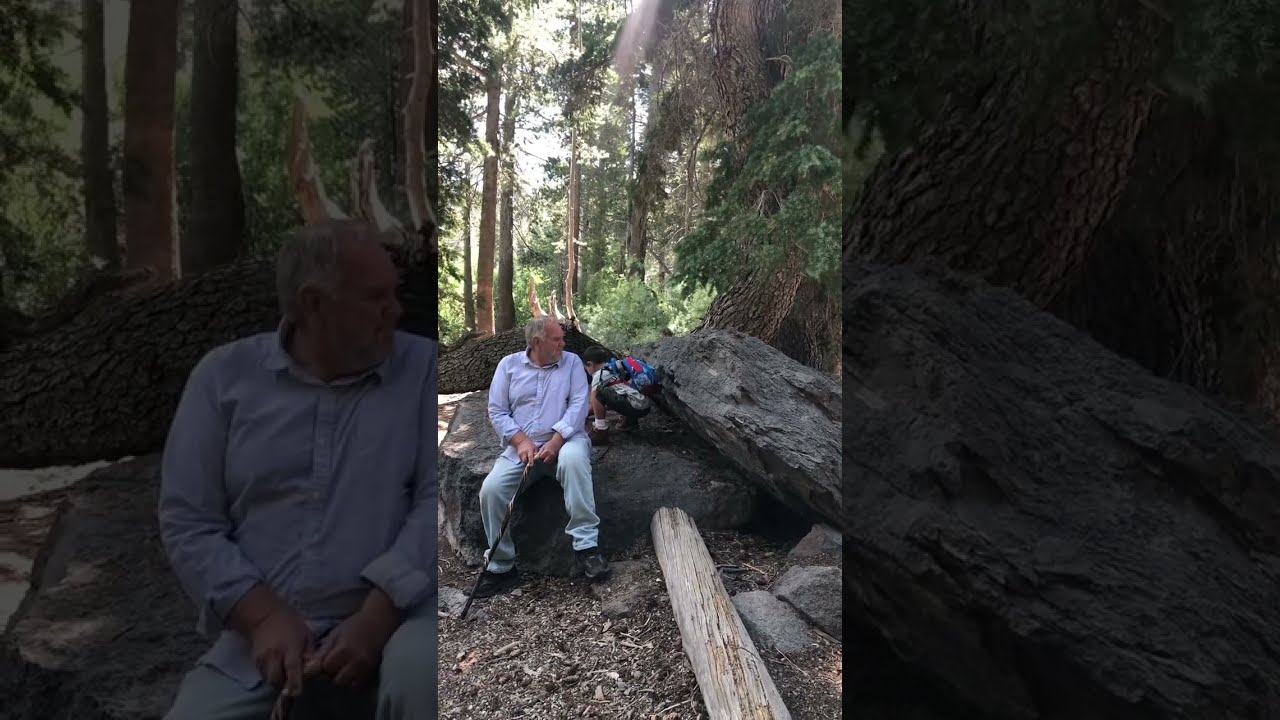A detailed caption for the image, incorporating shared elements and key details from all inputs:

An older man, possibly in his 50s, with slightly balding gray hair, sits on a large charcoal gray boulder in a wooded clearing. He wears a long-sleeve white button-up shirt, blue jeans, and brown shoes. A long black cane rests in his hand. To his right, a young boy, around four or five years old and wearing a small backpack, leans down intently over the rock as if picking something up. The boy is bending forward with curiosity, while the man glances over his shoulder towards the child, his expression suggesting attentive care.

Surrounding them are several large gray rocks, one of which is propped against the boulder the man is seated on. Beneath them, the ground is littered with dried foliage, twigs, and small brown branches. A wooden log extends from the ground towards the rocks, and nearby, a long tree trunk rests on the ground. Towering redwood trees encircle the scene, their tall trunks and green canopy complementing the shaded yet sunlit ambiance. The sunlight filters through the trees, providing a soft glow to the otherwise shaded area.

Unique to the photograph’s artistic presentation are two zoomed-in overlays on either side of the main image: the right side shows a close-up of a portion of the boulder, while the left side features a close-up of the man from the waist up, subtly darkened by a black opaque overlay. This layered composition adds depth and artistic flair to the tranquil moment shared between the man and the child in the midst of nature.